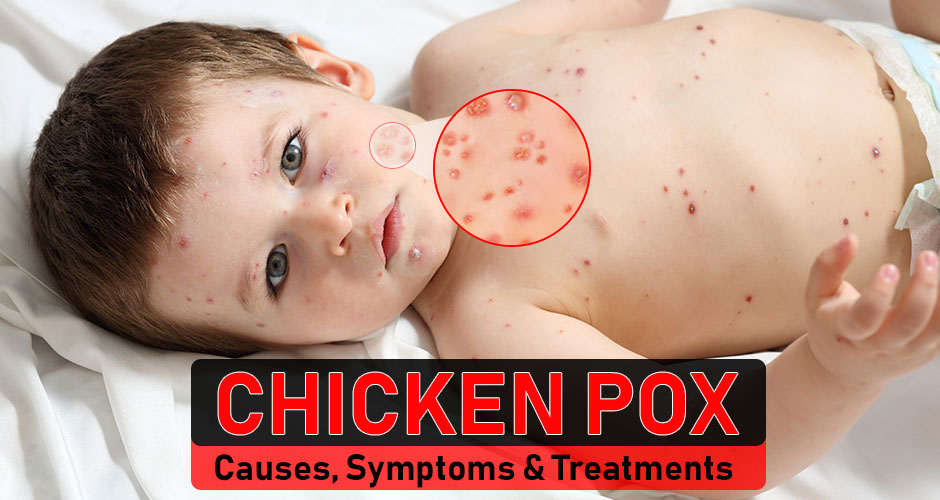The image depicts a young toddler with pale skin and short reddish-brown hair, laying sideways on a white sheet. His head is positioned to the left of the frame and his chest to the right, where his white diaper is just visible. He is looking directly at the viewer with grayish eyes. The child’s body and face are covered in small, scabbing, and crusty chickenpox pustules. Some of the sores are starting to peel, particularly one on his chin that is turning white. A red circle highlights a close-up view of the pustules, showing their detailed appearance with red edges and white pus-filled centers. At the bottom of the image, bold red capital letters spell "CHICKEN POX," with a thin white outline, on a black background. Below this, a red rectangular section with black letters lists "CAUSES, SYMPTOMS, AND TREATMENTS."